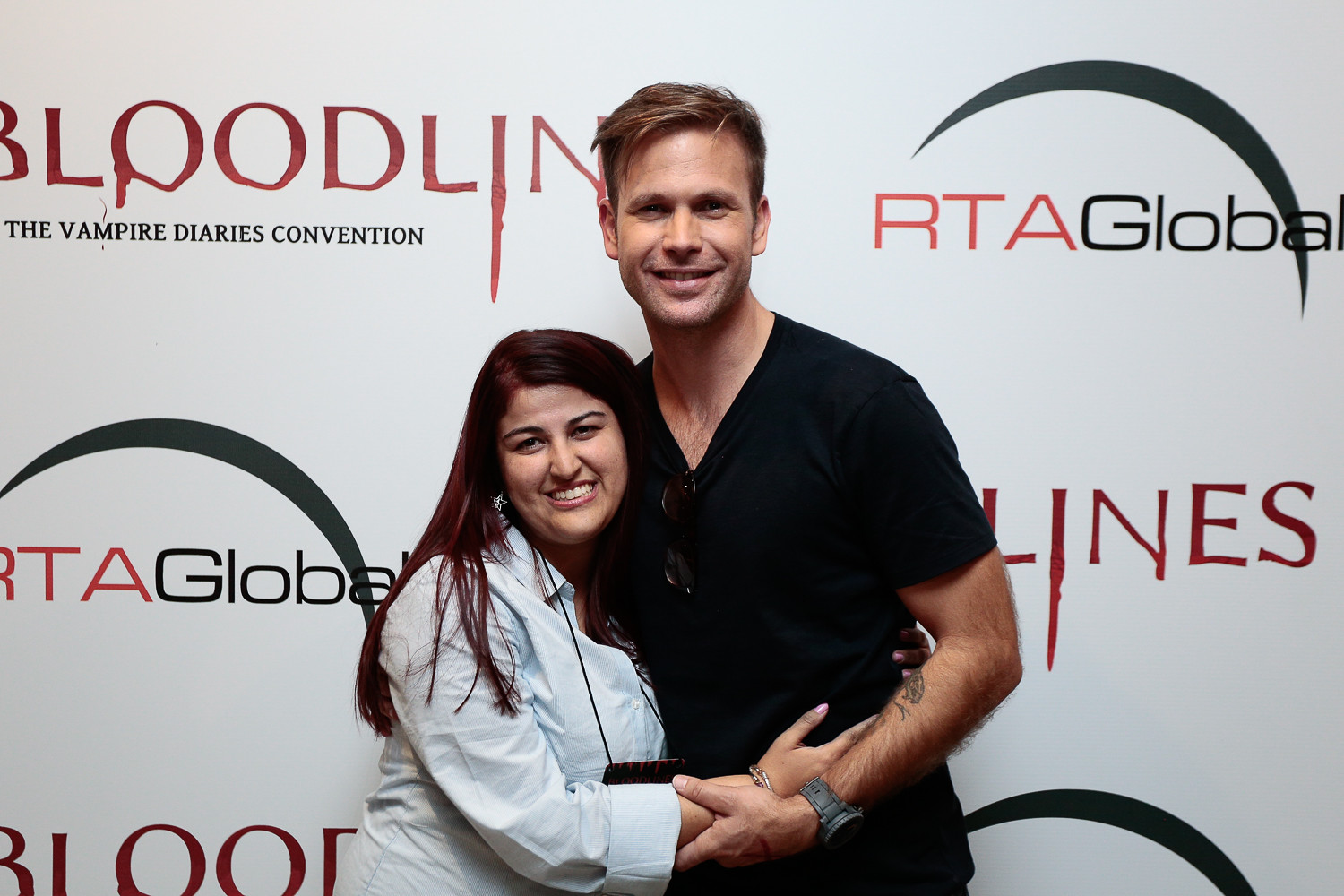In this image, a man and woman are posing in front of a white backdrop adorned with patterned writing and logos. The prominent logos include a red "Bloodline" and the black "The Vampire Diaries Convention" beneath it, as well as another logo with a black arch over black and orange text reading "RTA Global."

The woman stands on the left, smiling warmly at the camera. She is dressed in a long-sleeved, light-colored collared shirt and has burgundy hair cascading down her back. Although partially obscured by her arm, she appears to have some small item hanging from her neck, likely her cell phone. She has her arm around the waist of the man beside her.

The man, significantly taller by about a foot, is positioned on the right. He is also smiling, wearing a black v-neck shirt with dark sunglasses hanging from the neckline, and a gray watch on his wrist. He possesses a tattoo on the inside of his forearm. They both have their arms around each other, facing the camera against the distinct backdrop, creating a warm and engaging portrait.